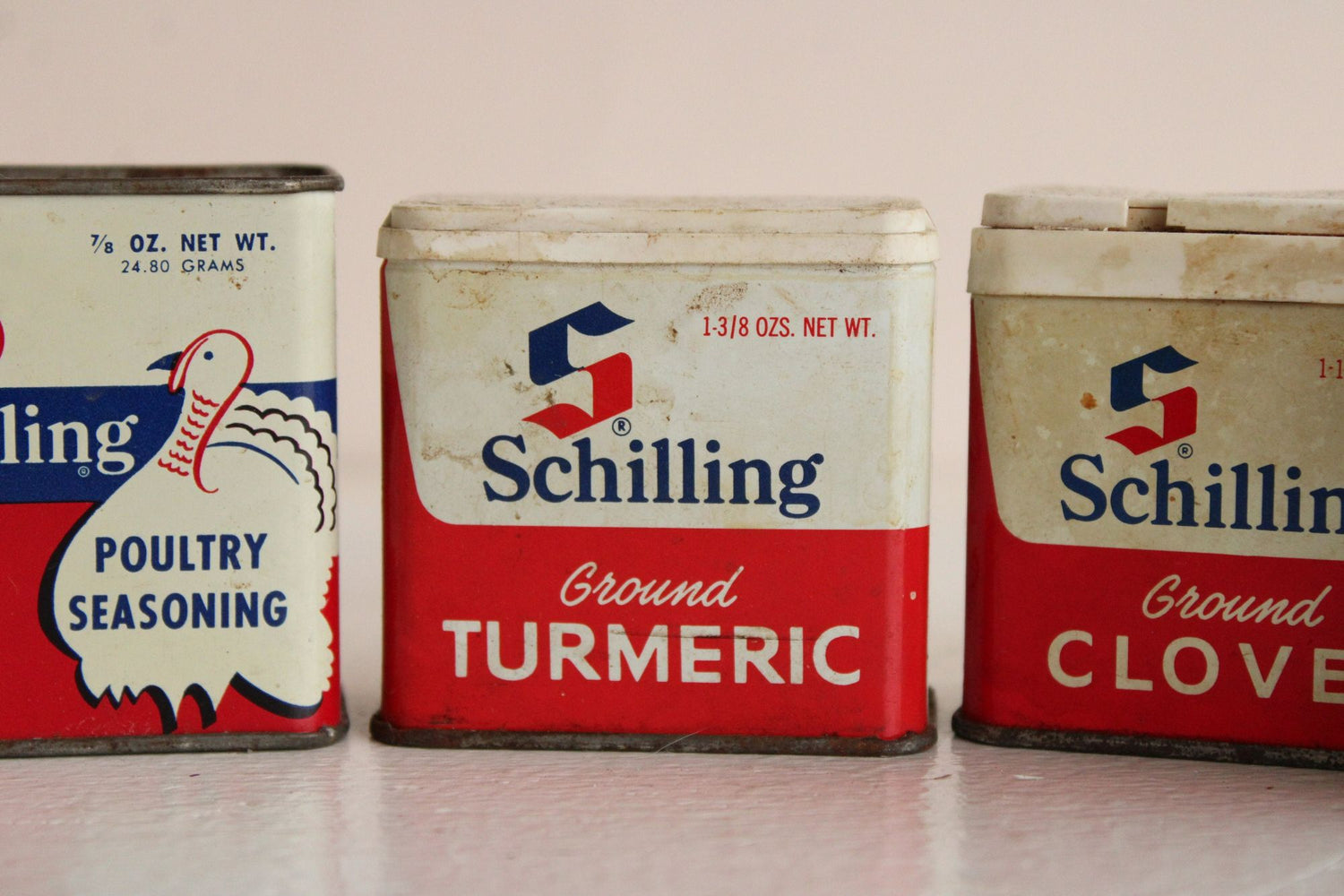The image is a landscape-oriented color photograph showcasing three vintage tins of seasonings, placed side-by-side and facing the viewer. Each tin displays a red, white, and blue motif with distinct graphics. On the left is an antique Poultry Seasoning tin, prominently featuring an illustration of a chicken and the text "Poultry Seasoning" in dark blue. This tin is white, red, and blue, and specifies a net weight of seven-eighths ounce (24.80 grams). 

In the center, the tin for Schilling Ground Turmeric stands out with its rusty top. It has a white upper section with the Schilling logo—an S in red and blue—and the brand name in dark blue. The lower section is red with "Ground Turmeric" printed in white letters.

On the right is another Schilling tin, this one for Ground Cloves. Similar in design to the turmeric tin, it also features the Schilling logo and branding, along with "Ground Cloves" in white text against a red background. This tin is noticeably dirtier compared to the other two. Overall, the photograph captures the vintage and well-used character of these spice tins with a style that emphasizes photographic realism.